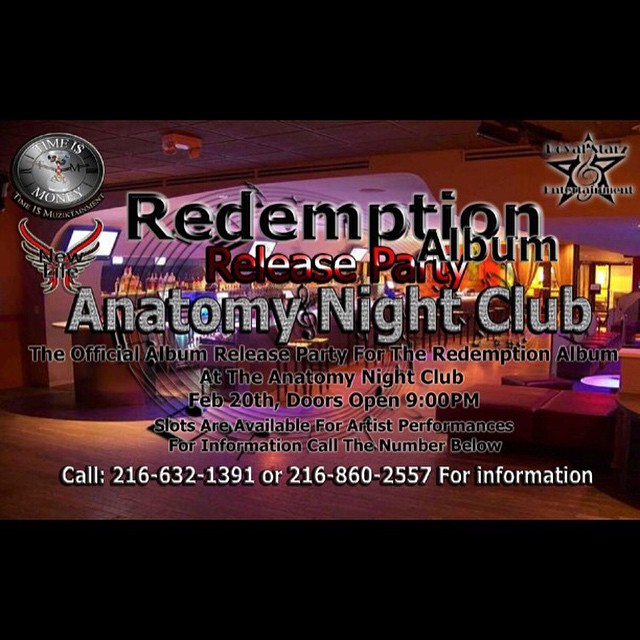The image is a busy, slightly disorganized advertisement for an album release party at a nightclub. At the top, it prominently features the text "Redemption Release Party Album," followed by "Anatomy Nightclub" written in a font that appears to be designed with diamonds. Beneath that, it reads, "The official album release party for the Redemption album at the Anatomy Nightclub, February 20th, doors open 9 p.m. Slots are available for artist performances. For information, call 216-632-1391 or 216-860-2557." On the left-hand side, there is a clock logo with the text "Time is Money," and nearby, a smaller image with the words "New Life" written on it. In the upper right, there's a star with illegible text inside. The overall layout includes black borders on the top and bottom, creating a rectangular frame around the elements.